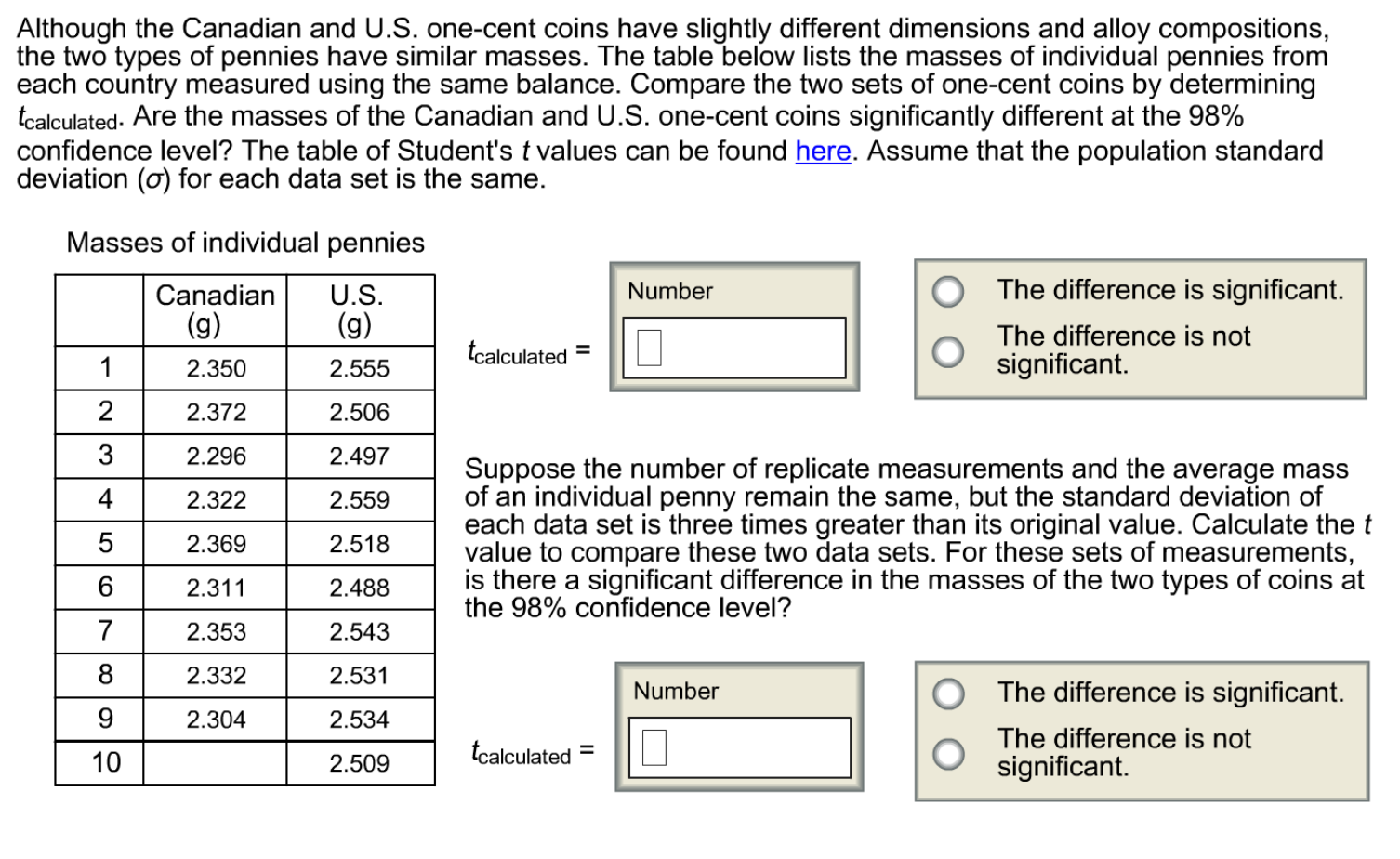The infographic depicts a detailed comparison between Canadian and U.S. one-cent coins, specifically focusing on their masses. Arranged in a rectangular table wider than it is tall, the comparison includes ten rows numbered 1 through 10. Each row lists the mass of a Canadian penny in grams alongside the mass of a U.S. penny in grams. Above the table, a header reads: "Although the Canadian and U.S. one-cent coins have slightly different dimensions and alloy compositions, the two types of pennies have similar masses."

In addition to the table, there's a calculator feature with a beige interface that allows users to input the masses. These entries will determine if the difference between the two coin types is significant or not, based on user selections. Below these input fields, a paragraph provides additional context, explaining that the table lists the masses of individual pennies measured using the same balance and that users are to determine if the differences are statistically significant at the 98% confidence level. The calculator is interactive, designed to aid in this comparison by calculating the difference once the user inputs the masses.